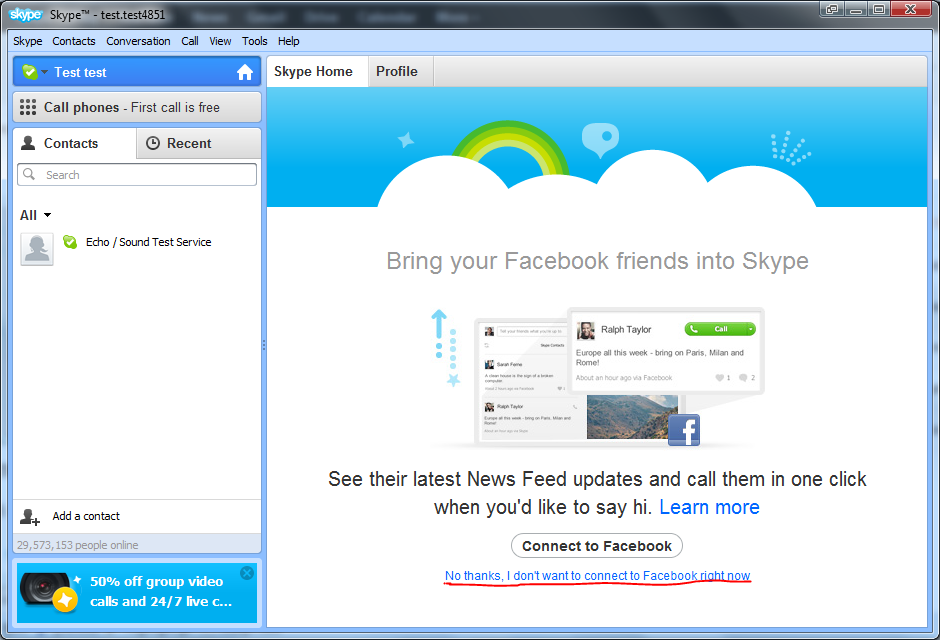This is an image from a Skype profile on the Skype website. At the top, the word "Skype" appears in blue letters against a white background. Below, "Skype™" is written in black letters followed by "— test.test4851". The menu bar includes clickable sections labeled Skype, Contacts, Conversation, Call, View, Tools, and Help. Directly beneath this, the text "Test, Test" is displayed.

Centered on the page, there are options for "Skype Home" and "Profile". On the left, under "Test, Test", there is an option labeled "Call Phones", which mentions that the first call is free. Additional options include "Contacts" and "Recent". A search bar allows users to find contacts, including the "Echo / Sound Test Service". At the very bottom, a button labeled "Add Contact" is present, next to a notification that there are currently 29,573,153 people online. 

A promotional banner at the bottom advertises "50% off group video calls and 24-7 live support" with an image of a camera icon. In the center of the page, the text encourages users to "bring your Facebook friends into Skype" alongside a Facebook symbol. A sample conversation between two users, Ralph Taylor and another person, highlights a message saying "You're up all this week. Bring on Paris, Milan, and Rome." with a green "Call" button.

Below this sample conversation, a message invites users to see their friends' latest newsfeed updates and to call them with one click. Options to "Learn More" and "Connect to Facebook" are given, with an additional option "No thanks, I don't want to connect to Facebook right now" crossed out with a red line.

The entire layout is set against a white background, accented by clouds, a greenish-yellow rainbow, and an overall blue background.